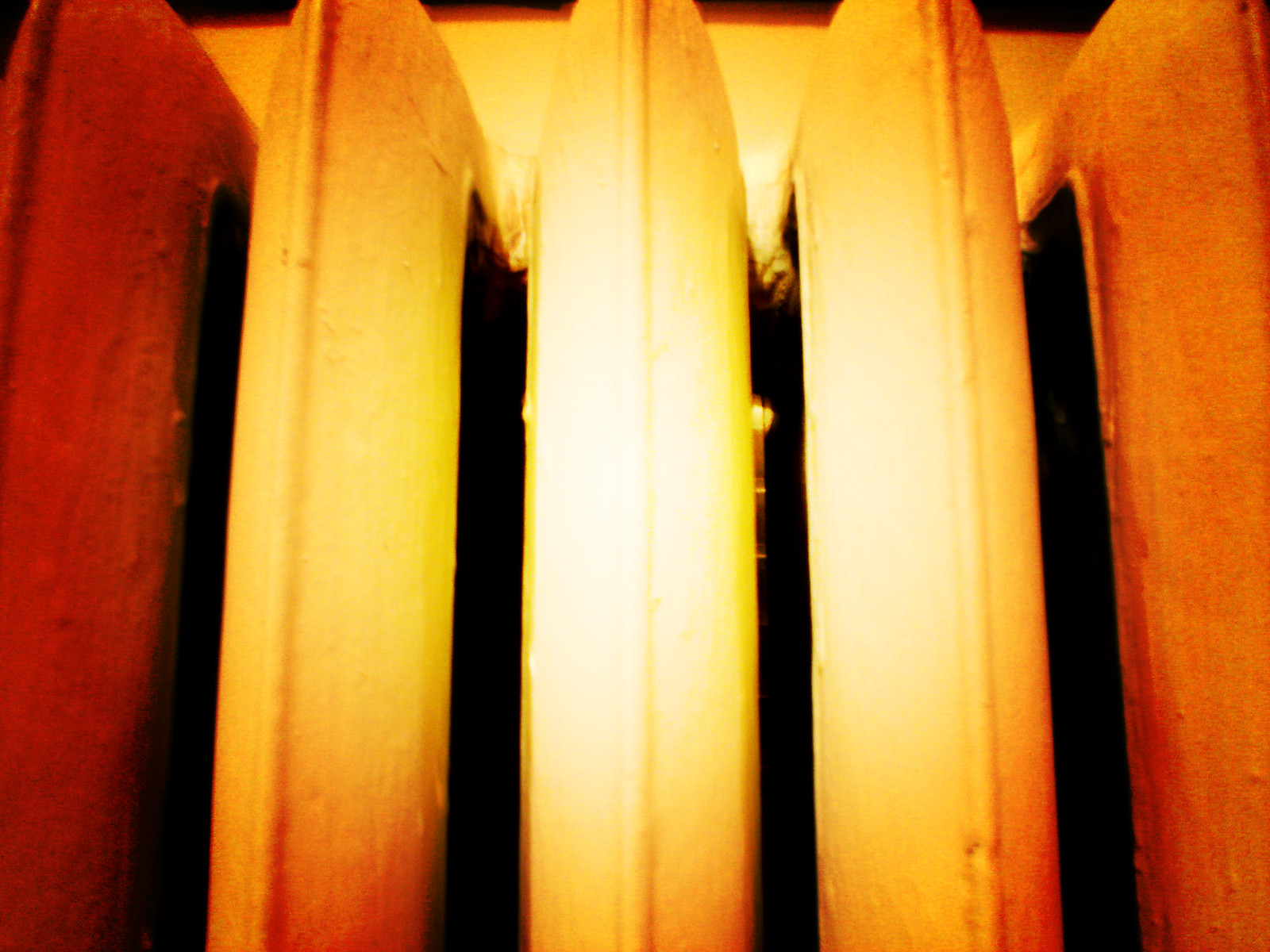This image is an extreme close-up of an old-style steam radiator, commonly found in New York City apartments and historic buildings. The focus is on five metal pipes or vents made of iron, which are traditional components of this type of heater. These pipes are designed with spaces between them to allow heat to escape efficiently. The lighting in the image is quite unique, with the center vent illuminated by a warm white light, creating a bright highlight that gradually fades into a dimmer, warmer light towards the edges. Due to the lighting and close-up nature of the shot, it's challenging to discern the exact color of the radiator, which appears to be either white or beige.